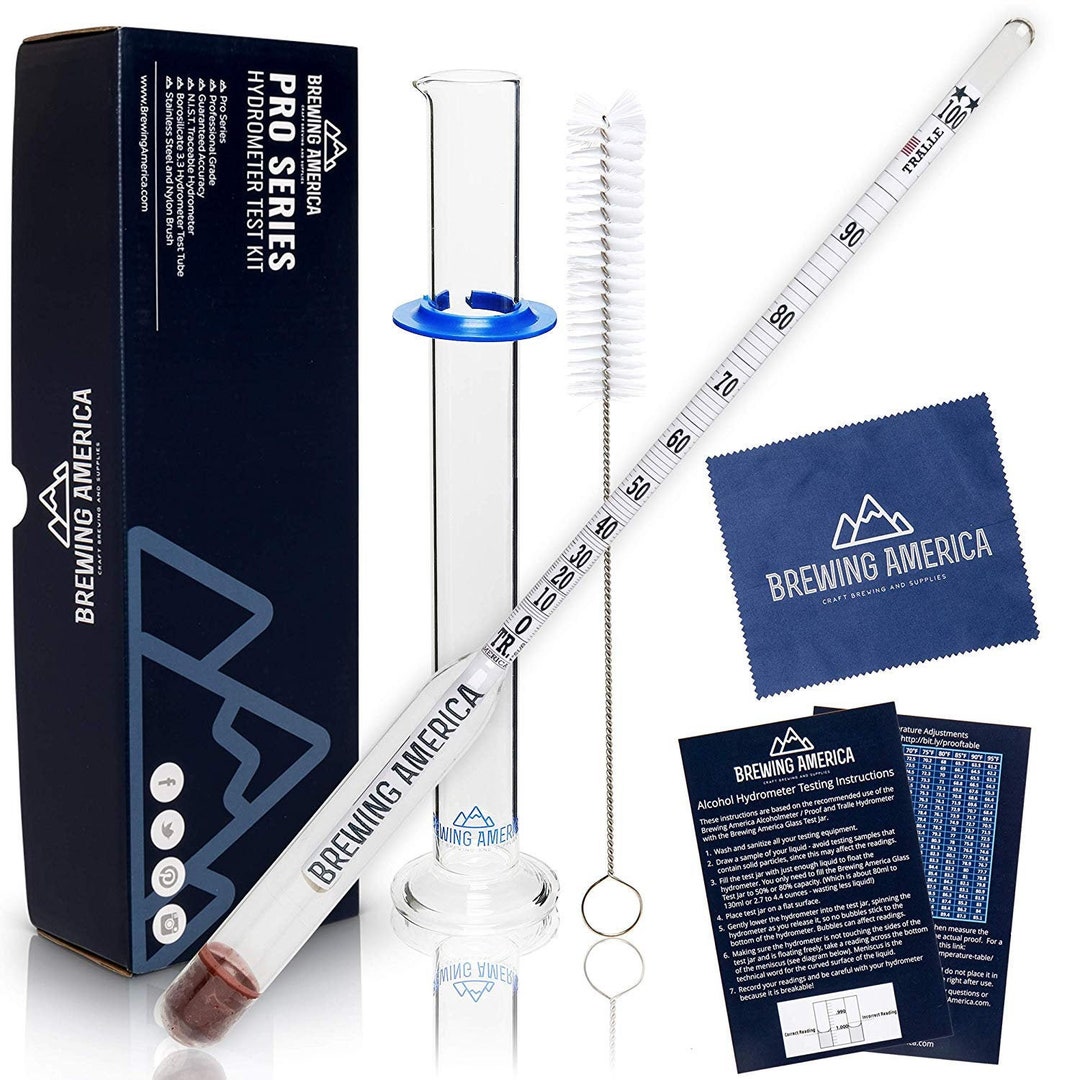This image showcases a comprehensive stock advertisement photo for the Brewing America Pro Series Hydrometer Test Kit, set against a pristine white background. On the left side of the image stands the sleek black packaging, adorned with white text that reads "Brewing America Pro Series Hydrometer Test Kit." The sides of the box prominently display the "Brewing America" branding along with an enlarged blue-grey emblem of their signature Three Mountain logo, which unveils graceful snow-capped peaks.

Laid out meticulously to the right of the packaging are the contents of the kit: a glass test tube boldly labeled "Brewing America," a long, detailed thermometer with the same branding, featuring numerous graduations and numerals ranging from 10 to 100. Nearby, a sturdy brush with white bristles hints at maintenance and precision. Two black pamphlets feature detailed text, charts, and the recognizable Brewing America logo, positioned adjacent to a small, neatly folded piece of cloth that bears the Three Mountain emblem and the company name.

The array of items is complemented by visual aids, including what seems to be a key to understanding the thermometer's graduations. This well-organized display emphasizes the professional and meticulous nature of Brewing America's hydrometer test kit, appealing to brewers who value both function and presentation.